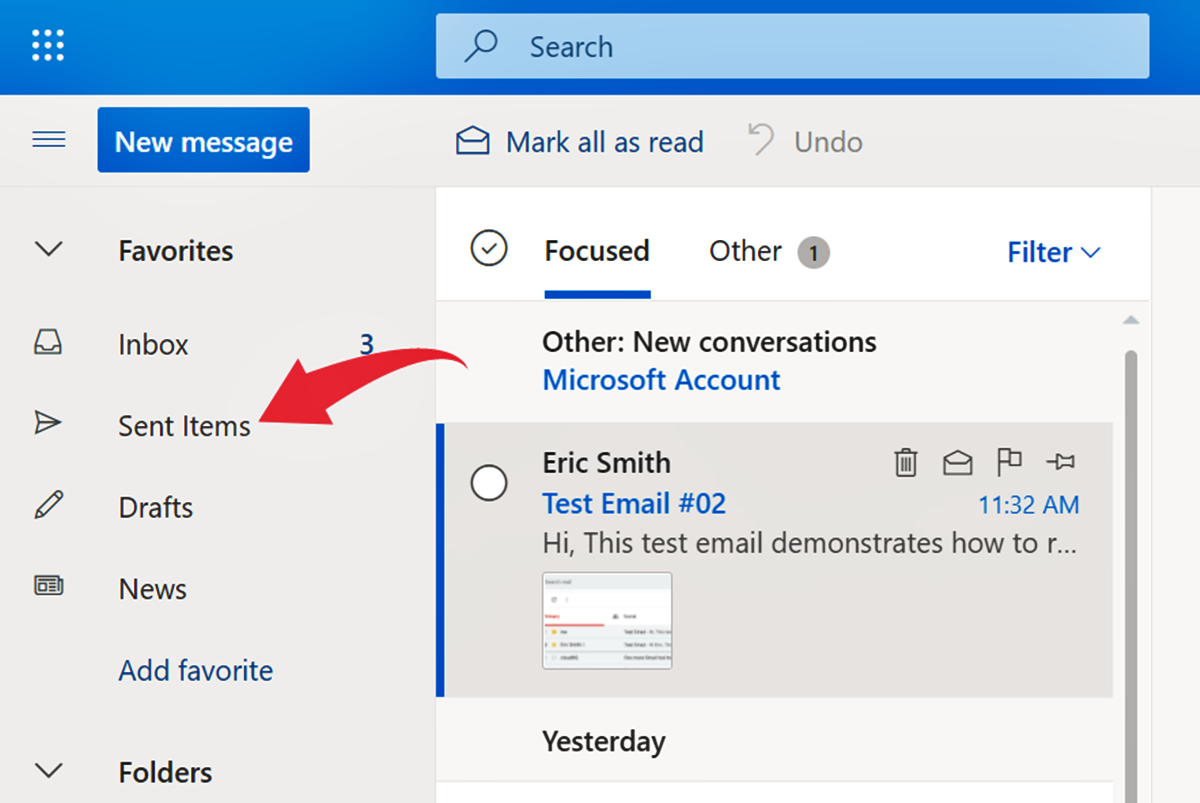The image depicts a computer screen showcasing an email system interface. At the top of the screen, there is a search bar. Beneath it, a blue rectangular box spans the width of the screen, likely indicating the currently selected email category. Various categories are organized in a list, including "New Message," which is highlighted with a blue rectangular box as well.

Moving downwards, the "Favorites" section is visible with subcategories such as "Inbox" and "Sent Items." The "Sent Items" category is specifically highlighted with a red arrow pointing towards it. Inside this arrow is a white box containing a circular checkmark icon, emphasizing its importance. The "Focused" tab is underlined next to the word "Other," and these are followed by a "Filter" menu option with a dropdown arrow. Below, it reads "Other: New Conversations."

Within the "Sent Items" section, a selection labeled "Microsoft Account" is visible. The "Inbox" category shows three emails. Below the "Sent Items" are additional categories: "Drafts," "News," and an option to "Add Favorite." Further down is the "Folders" section.

To the right, the interface lists the emails and their details. There is an option to "Mark All as Read." One of the visible emails, titled "Eric Smith - Test Email Number Two," includes the preview text, "Hi, this test email determines how to..." and is timestamped "Yesterday."